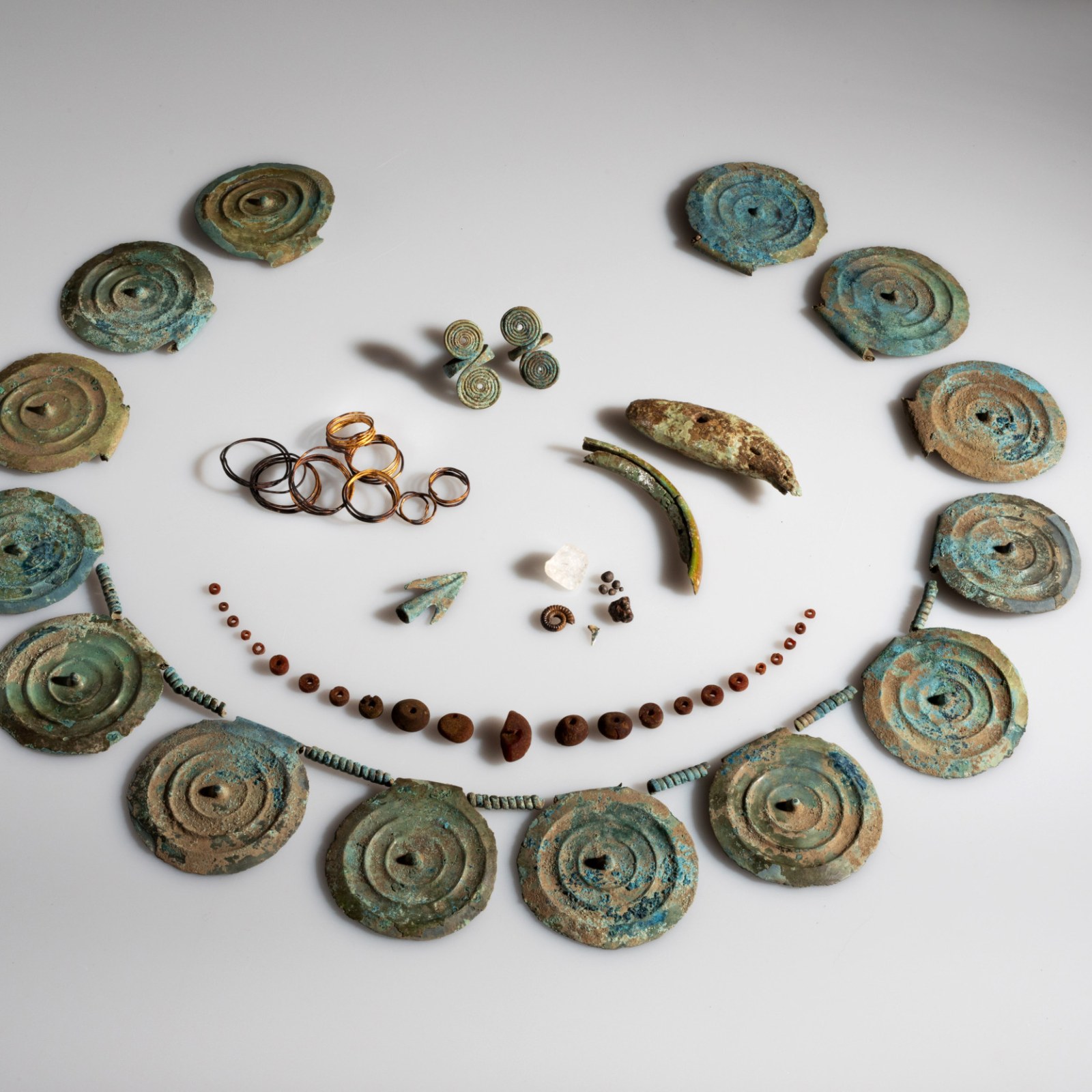This is a detailed color photograph on a white background showcasing what appears to be very old, possibly ancient, jewelry that looks like it was excavated from the ground. The items are arranged in a semicircular pattern and include a variety of circular metallic pieces that have a turquoise coloring with rust or corrosion. These pieces exhibit intricate designs with small dots and circles radiating from their centers. Prominently featured are several copper-colored discs with a green patina, suggesting significant age and exposure to the elements. Below these discs, arranged in the shape of what might have been a necklace, are dark brown or maroon stone beads alongside gold or bronze hammered rings. An arrowhead and various pebbles are also part of the collection, along with wire rings and what possibly could have been earrings, characterized by circles at the top and bottom. The image casts shadows that add depth to these ancient artifacts, each telling a story of a bygone civilization.